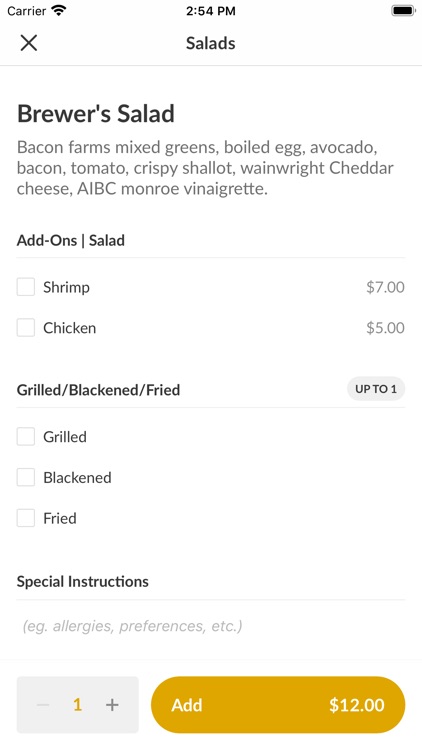Screenshot of an online salad order interface displayed on a mobile phone. The layout is in portrait orientation, distinctly taller than it is wide. The image features a white background with no visible borders. The uppermost section displays the mobile carrier's details, Wi-Fi signal, and battery icon, indicating it is 2:54 p.m. Below this, there is a thin gray underline spanning the width of the screen.

The main content begins with the title "Brewer's Salad" in the largest, boldest font on the page, followed by a detailed description in smaller, left-justified text that spans approximately three lines: "bacon, farms mixed greens, boiled egg, avocado," and continues.

Beneath this, still left-justified, is a section labeled "Add-Ons" in bold, smaller font, indicating options for additional ingredients. Two clickable light gray boxes are aligned below this section. The first option is "Shrimp" priced at $7.00, and the second is "Chicken" priced at $5.00, both unselected.

Further down, there's another category for preparation style: "Grilled / Blackened / Fried." The right corner features a gray oval stating "UP TO ONE" in uppercase darker gray font. Below this is a selection area with three unclicked boxes labeled "Grilled," "Blackened," and "Fried."

The final section is titled "Special Instructions" in smaller, bold font. It has a thin underline and a placeholder text in light gray italics that reads "(e.g. allergies, preferences, etc.)"

At the bottom of the screen, there's a horizontal gray rectangle which includes an orangish-brown button for selecting the quantity of salads, flanked by a grayed-out minus sign on the left and a darker plus sign on the right. To the right of this, a larger orangish-brown button displays "Add - $12.00" in white font on the left and right sides respectively.